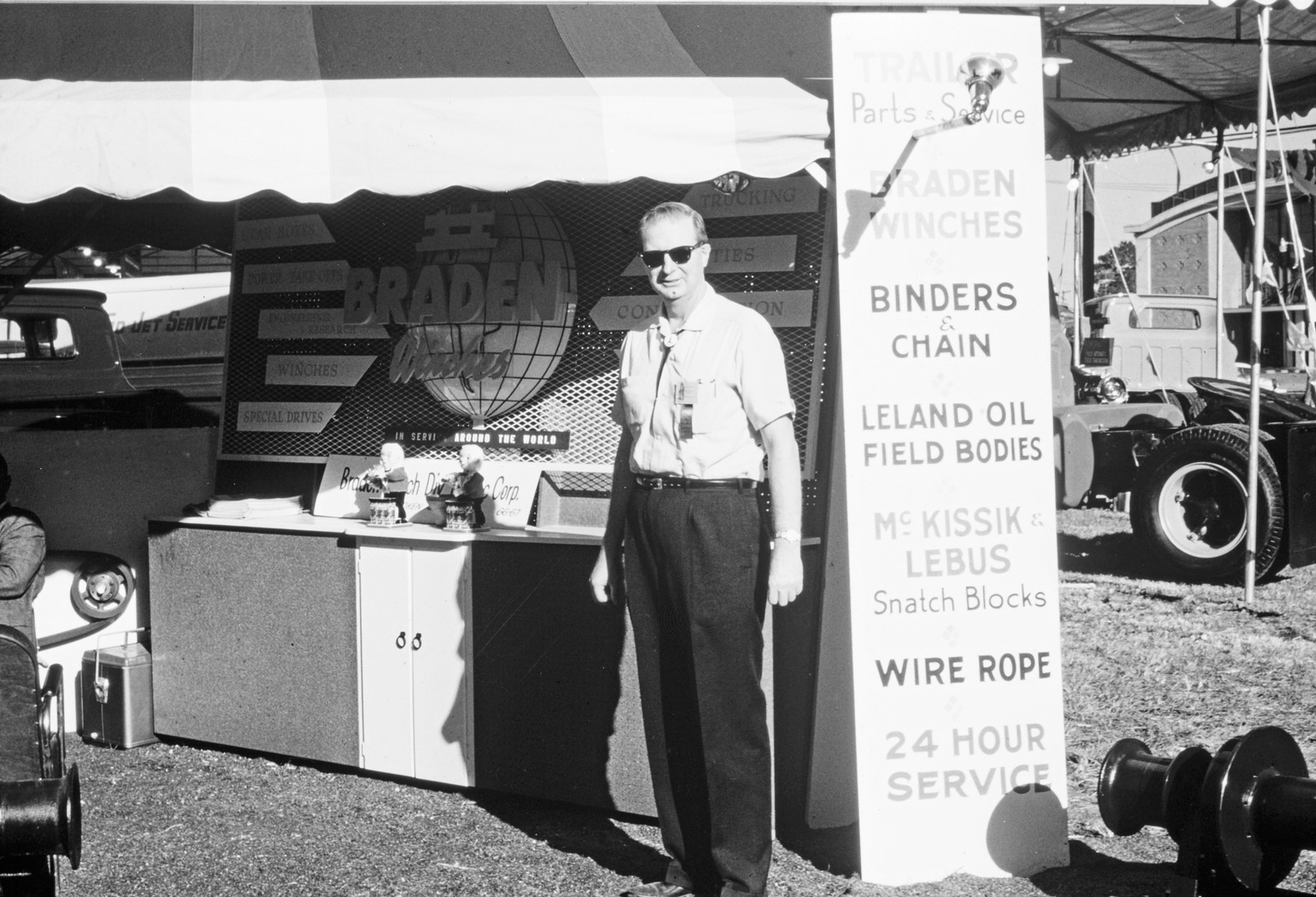This black and white photograph captures an older man, likely in his 50s or 60s, standing under a striped tent on a sunny day, possibly at an automobile or trade show event in the 1950s. The man, a white male, is dressed in sunglasses, a white business shirt, and black pants, and he is posing in front of a booth dedicated to Brayden winches and related services. A large, prominent sign next to him, taller than he is, lists various offerings such as trailer parts and service, Brayden winches, binders and chain, Leland oil field bodies, McKissick Libus snatch blocks, wire rope, and 24-hour service. Equipment and automobile parts are scattered around the tent, with a counter displaying items that are unclear, possibly including two bobbleheads. The booth features backboards with the word "Braden" and other related specialty services, suggesting that Brayden winches is the main company sponsoring this demonstration booth.